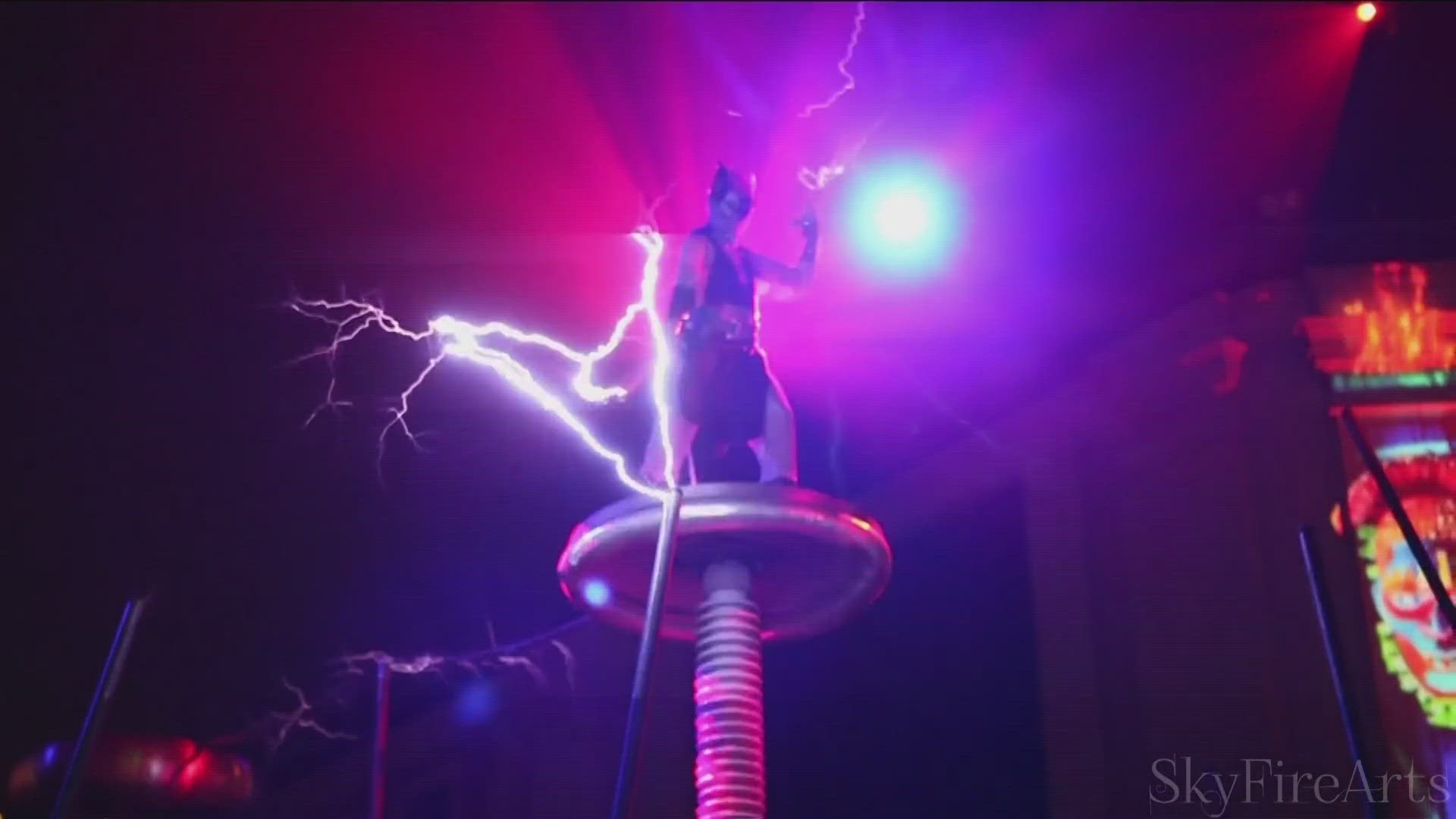The photograph captures a striking scene featuring a man who appears to be a performer standing on a silver, metallic pedestal, likely a high-voltage platform. His wild hair and dramatic face mask create an imposing presence. He is dressed in a tunic or kilt with white pant legs extending below and a dark vest. A large, bright light, possibly blue, shines above him, casting a surreal, purple-reddish hue over the entire scene. Lightning bolts erupt from his right hand, seemingly emanating from an electrode or a Van de Graaff generator near the base of the pedestal, sending electrical currents in all directions. His left arm is also raised as if in mid-performance. The backdrop is dim, particularly in the left-hand corner, which features a dark entranceway, while to the right, an object that resembles an arcade game is partially visible. In the top right corner, a yellow circle projects rays of red light. The photograph, marked with a watermark at the lower right that reads "Skyfire Arts," has elements that are slightly blurred, adding to the dramatic and mystical atmosphere.